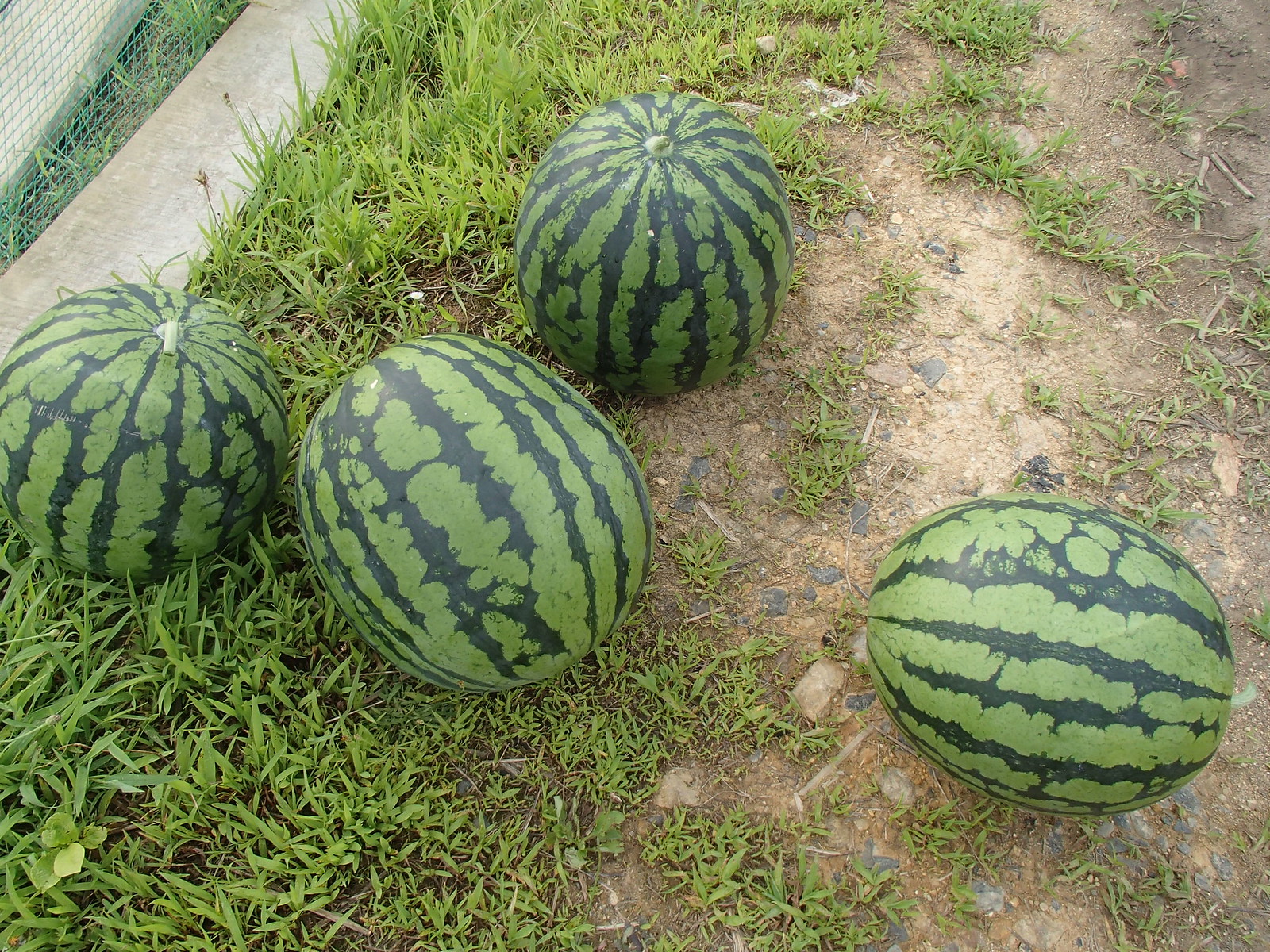This color photograph captures four perfectly shaped watermelons resting on the ground. The watermelons, with their light green skin adorned with darker green stripes and a net-like pattern, are positioned in an earthy setting. Three of the watermelons are clustered together: two sit upright, showcasing their stems, while the third one lies on its side. The fourth watermelon sits alone on the right side of the image, also lying on its side. The ground they rest upon is a mix of bare earth, scattered rocks, and patches of grass. In the top left corner, the bottom portion of a fence or a piece of plywood with some fencing can be seen, adding context to the setting. The area beneath the watermelons near the fence has thicker grass, suggesting it is a spot less traveled.